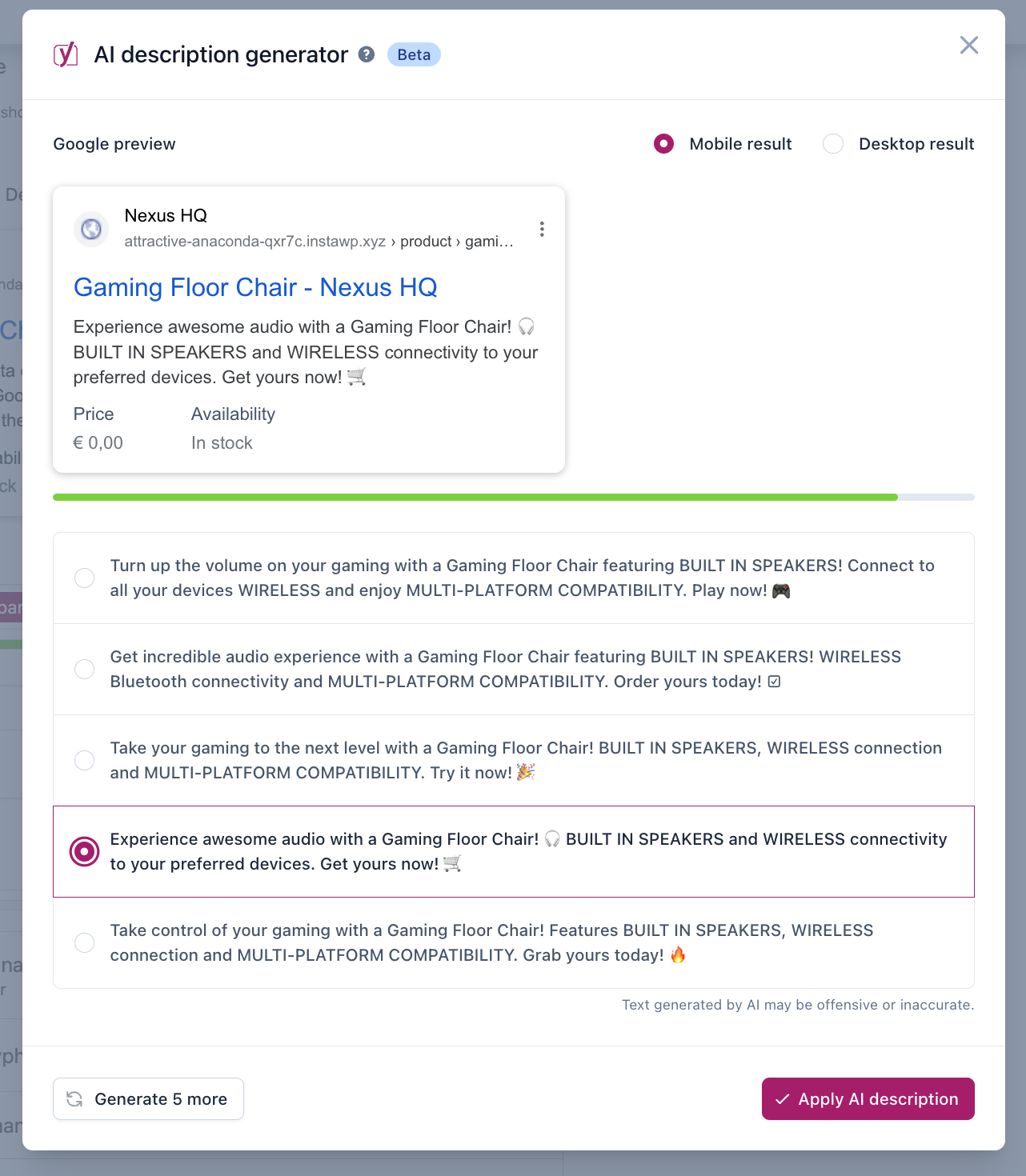Displayed on the website is an AI description generator tool, showcasing a product description example. Beneath the generator interface, there's a Google preview of the product listing. The small white window highlights the Nexus HQ gaming floor chair. The description emphasizes its immersive audio experience, featuring built-in speakers and seamless wireless connectivity to various devices. The promotional offer states the chair is available for €0, with immediate availability in stock.

Below the description, five button options are clearly presented. Adjacent to these buttons on the left are light gray circles, each preceding a concise two-sentence text snippet generated by the AI. In the bottom right corner, a prominent purple button with white text invites users to "Apply AI Description." On the left-hand side of the interface, there's an option to generate five more description variations.

The layout suggests this tool is explicitly designed for creating detailed and appealing product descriptions, with the current focus being on the Nexus HQ gaming floor chair, offering potential selections from five AI-generated options.